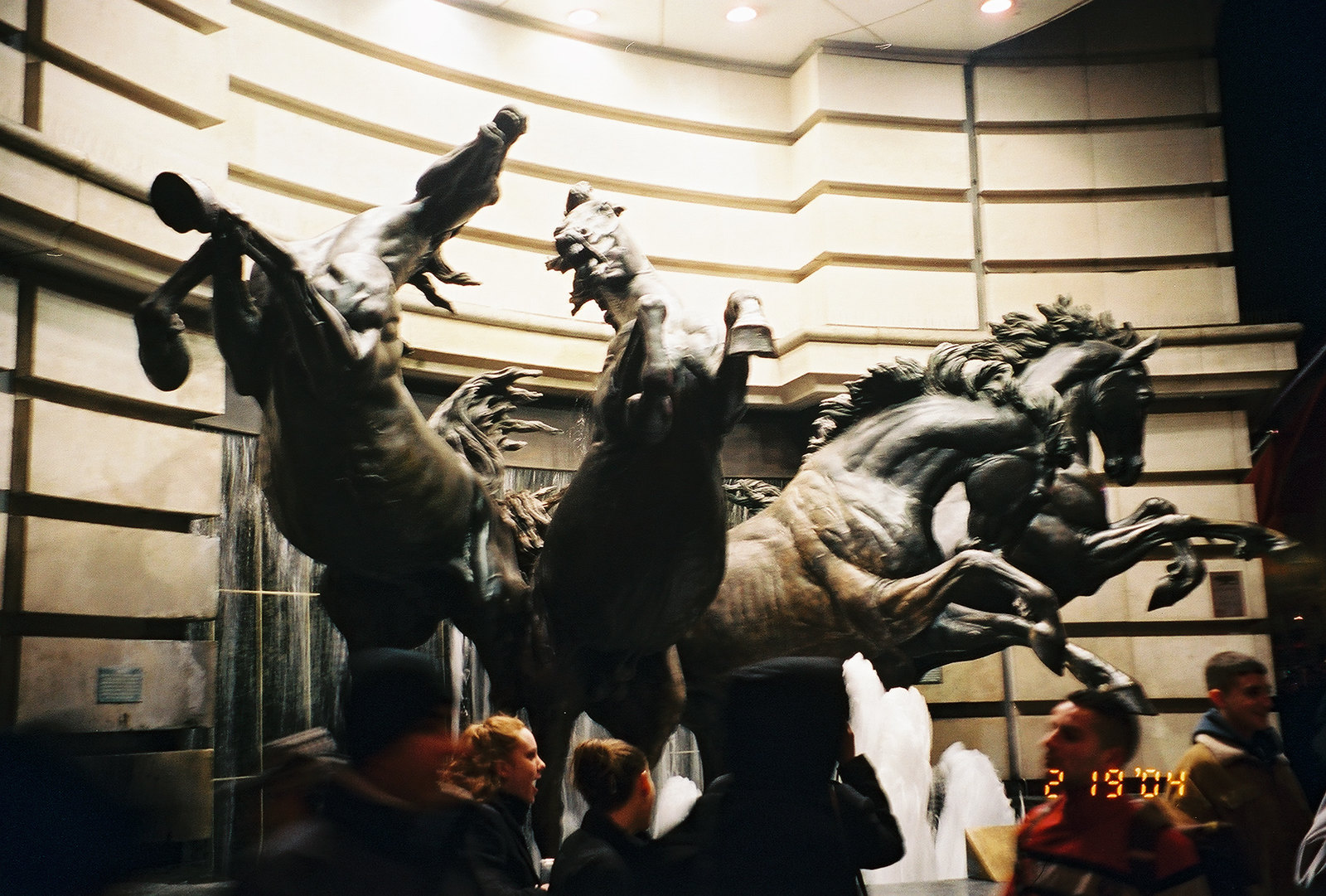The image depicts a striking nighttime scene centered around a dynamic metal sculpture of four stallions, captured in the midst of a fierce, aggressive pose with their front legs raised high, as if bucking. This dramatic arrangement of horses, heads tipped at various angles, serves as the main focal point. The photograph, characterized by a monotone palette of dark brown, black, and gray tones, also features a time stamp in orange letters reading "2-19-04" in the bottom right corner.

The scene is set outside, likely near a building, evidenced by the architecture in the background which includes a tan stone wall and a white overhang with recessed lighting. Just behind the horse sculptures, a window is visible, adding to the ambiance of the location. Below the statues, six or so individuals are engaged in casual interaction, some walking from left to right, while others are standing and observing the artwork. The overall composition of the image harmonizes the energetic posture of the stallions with the serene, milling crowd below, against the backdrop of intriguing, softly lit architecture.